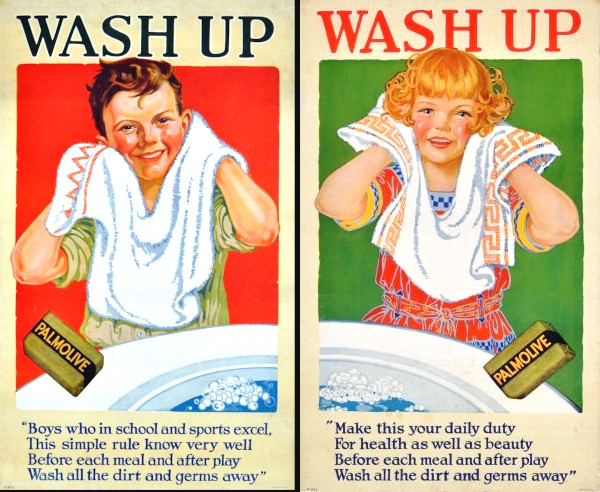The image features two advertisement posters for Palmolive soap, split in half to highlight their similarities and differences. 

On the left side, bordered in tan, the poster showcases a boy in a green short-sleeved shirt with brown hair and rosy red cheeks. He is depicted wiping his face with a white towel that has orange designs. In front of him is a white sink basin filled with blue water and white soap bubbles, within which floats a bar of soap tagged "Palmolive." Above him, bold black text reads "Wash Up," while at the bottom, blue text on the tan border reads, "Boys who in school and sports excel, this simple rule know very well: Before each meal and after play, wash all the dirt and germs away."

The poster on the right mirrors the left, set against a green background. It features a girl with yellow curly hair and rosy red cheeks, wearing a red dress with white, yellow, and blue accents, including a checkered collar and sleeves. She is holding a towel with orange and blue designs. Similarly positioned in front of a white sink basin with blue water and white soap bubbles, there is a bar of green soap. Red text at the top reads "Wash Up," with the caption at the bottom stating, "Make this your daily duty, for health as well as beauty: Before each meal and after play, wash all the dirt and germs away," in darker blue text.

Both posters emphasize the importance of hygiene with a consistent message to wash up before meals and after activities, appealing visually through vibrant and complementary designs.